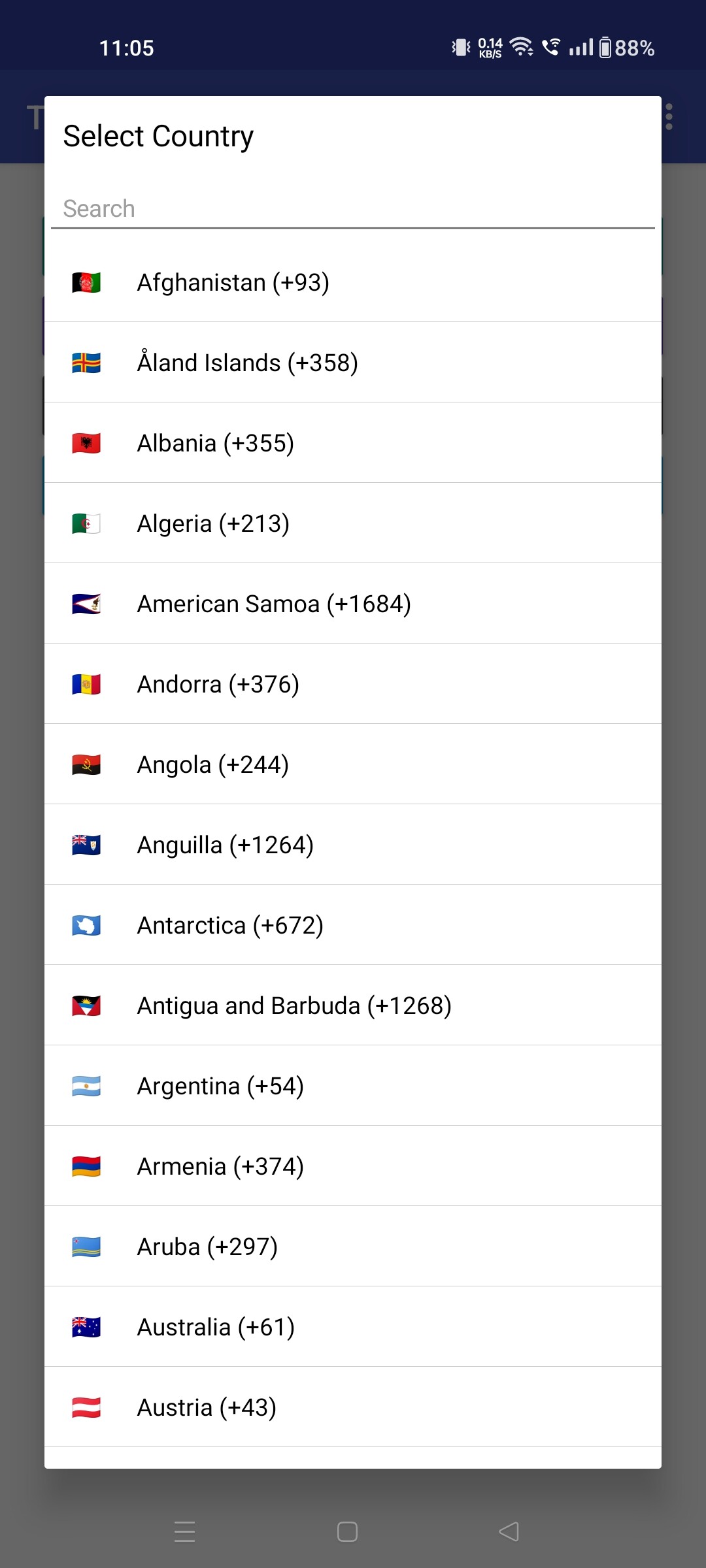On a smartphone screen, a white overlay displaying a drop-down menu of countries appears prominently, with the option to search and select a country. The background, showcasing the device's main screen, features a blue header at the top indicating the time as 11:05, full Wi-Fi signal strength, a phone icon, full reception bars, and an 88% battery level. The white overlay lists countries alphabetically with each entry accompanied by the respective national flag in color on the left, followed by the country name and its international dialing code in a bracketed plus sign format. The visible section includes countries from Afghanistan (+93) to Austria (+43). Beneath the blue header, the background is light gray and the navigation bar with three buttons is at the bottom of the screen.